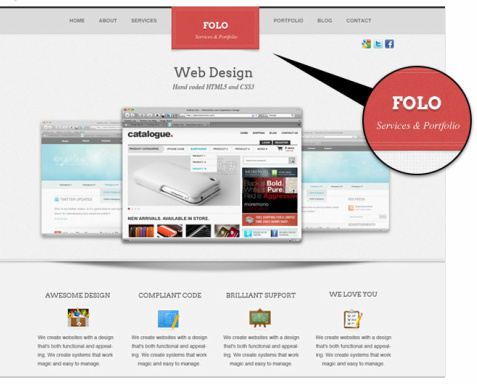This image is of a web design tutorial page, primarily featuring a gray and white color scheme. At the top is a navigation menu, all in capital letters, listing the following links: HOME, ABOUT, SERVICES, PORTFOLIO, BLOG, and CONTACT. Notably, the link to PHOTO, which falls between SERVICES and PORTFOLIO, stands out due to its bright red background color, distinguishing it from the rest of the menu.

On the right side of the menu bar are icons for social media platforms Google+ (now defunct), Twitter, and Facebook, allowing users to connect through these channels. Below the menu, the main content begins with a section prominently stating "WEB DESIGN - Hand-coded HTML and CSS3" in large text, emphasizing the website's proficiency in custom coding.

Beneath this headline, there are three example thumbnails of websites. One of the sites, labeled "Catalog," appears to showcase phone cases for sale. The details of the other two websites are less clear, showing light blue design elements and indistinct menu buttons.

Further down the page are four feature sections, each accompanied by an image and a brief descriptive paragraph:
1. **Awesome Design**: Accompanied by an image of a website layout, this section details the high-quality design services offered.
2. **Compliant Code**: Featuring an image of a blue square, this section explains the importance of adhering to web standards and best practices in coding.
3. **Reading Support**: Depicted with an image resembling either a TV or a chalkboard, this section highlights the supportive services available to clients.
4. **We Love You**: Illustrated with an image of a notepad and pencil, this section expresses the company's commitment to customer satisfaction.

Overall, the layout is clean and structured, providing a comprehensive overview of the web design services offered.